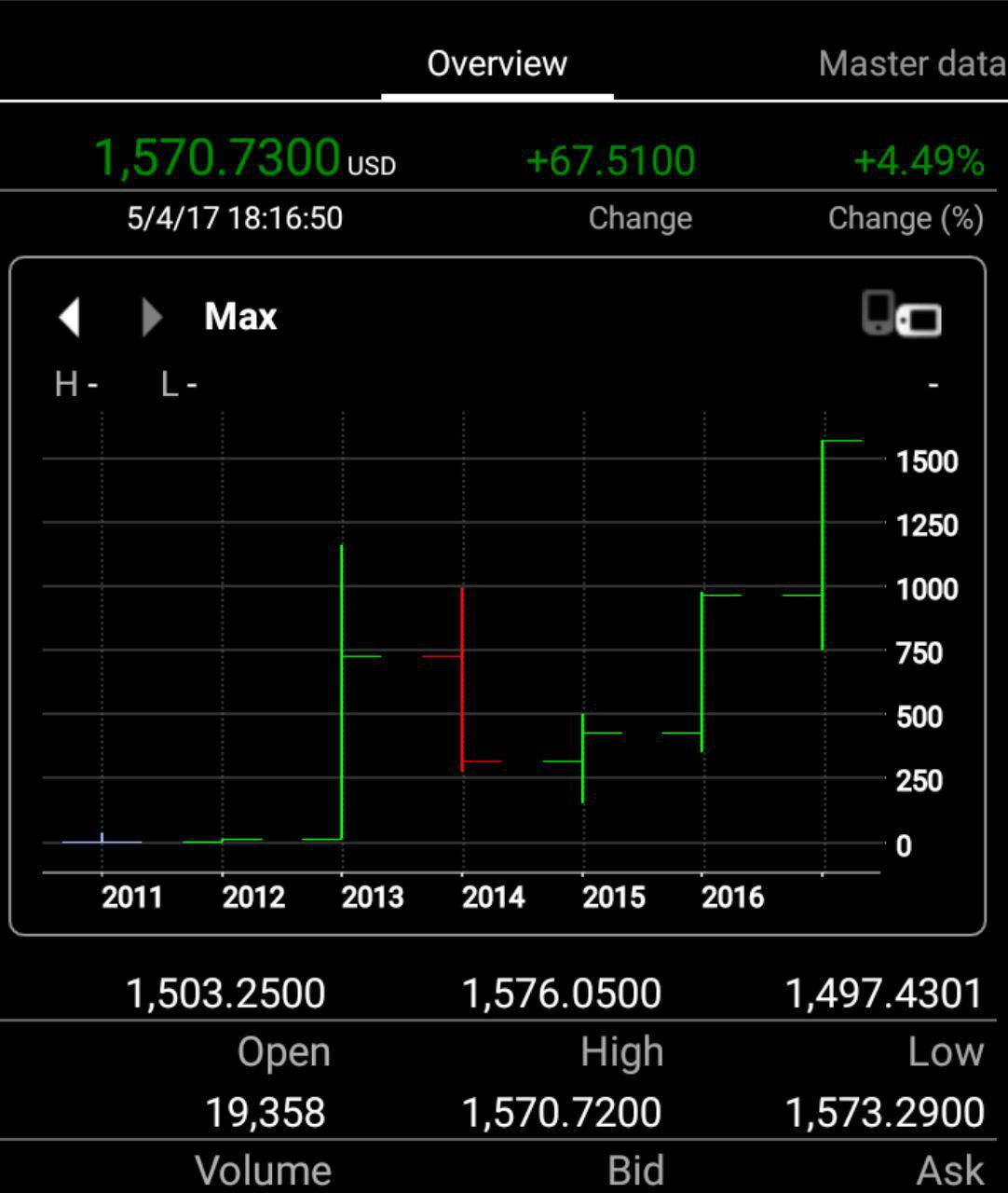Title: Detailed Financial Dashboard Display

Description: This vertical rectangular image showcases a sleek, information-dense financial dashboard against a completely black background. At the very center, the word "OVERVIEW" is presented in bold white font, accentuated with a thick white underline. Adjacent to it, on the right-hand side, "Master Data" is displayed in a light gray font. A white line spans across the entire heading area beneath these titles, while the thick underline specifically under "OVERVIEW" adds emphasis.

The following section features key financial metrics in vivid detail. Below "OVERVIEW," a green-font figure reads "1,570.7300" followed by "USD" in bold, capital white letters. Next, underneath "Master Data," a green-font displays "+6,7.5100" and "+4.49%." These figures are separated by a subtle gray line that horizontally crosses the image.

Further down, a timestamp "5/4/17 18:16:50" is prominently displayed in bright white font. The middle column houses the word "Change," and the right column displays "Change (%)" in parentheses.

The image also features a horizontal rectangular area outlined faintly in white. Located in the top left corner are two arrow icons, with the left-facing arrow bolded in white and the right-facing arrow in gray. To the right of these arrows, the word "Max" is written in bold white font. Additionally, the upper right corner contains several icons.

Dominating the center of the display is a graph, annotated at the bottom with years ranging from 2011 to 2016 in white bold font. The vertical axis runs from 0 to 1500, marked in increments of 250. The graph is further visualized with interlacing red and green lines.

Below the graph, respective bold white font figures include "1,503.2500" on the left, "1,576.0500" in the middle, and "1,497.4301" on the right. These are separated by a horizontal line.

The next row presents data points: "Open: 19,358" on the left, "High: 1,570.750" in the middle, and "Low: 1,573.2900" on the right. Another horizontal line follows beneath these values.

The final row lists "Volume" on the left, "Bid" in the middle, and "Ask" on the right. This meticulously detailed financial dashboard provides comprehensive insights, meticulously arranged for quick, actionable interpretation.